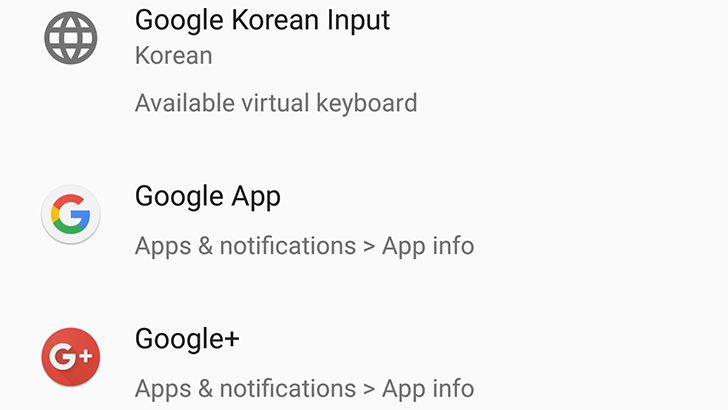The image is a detailed screenshot. On the right side, it features a square with a very pale light gray tone that becomes even paler on the left side, fading into a slightly darker gray on the right side. Overlaying the square, there is text and symbols. 

On the left side of the image, there is a small circle and two vertical lines aligned parallel to two horizontal lines, forming a grid-like pattern. Below these, two curved lines descend.

Adjacent to these symbols, the text reads "Google Korean Input" with capitalized first letters: 'G', 'K', and 'I'. Directly underneath, it says "Korean," followed by "Available virtual keyboard."

Towards the center of the image, there is another circle featuring the iconic Google 'G' in red, yellow, green, and blue colors. Next to this, it says "Google app" with the first letters 'G' and 'A' capitalized.

Beneath this section, the text "Apps and notifications" appears, followed by a right-pointing arrow, indicating a link to app information.

Further down, there is a red circle with a capital 'G' and a plus sign next to it. The text "Google+" is positioned outside this circle in black letters. Underneath it, once again, the text "Apps and notifications" is followed by a right-pointing arrow, denoting app information.